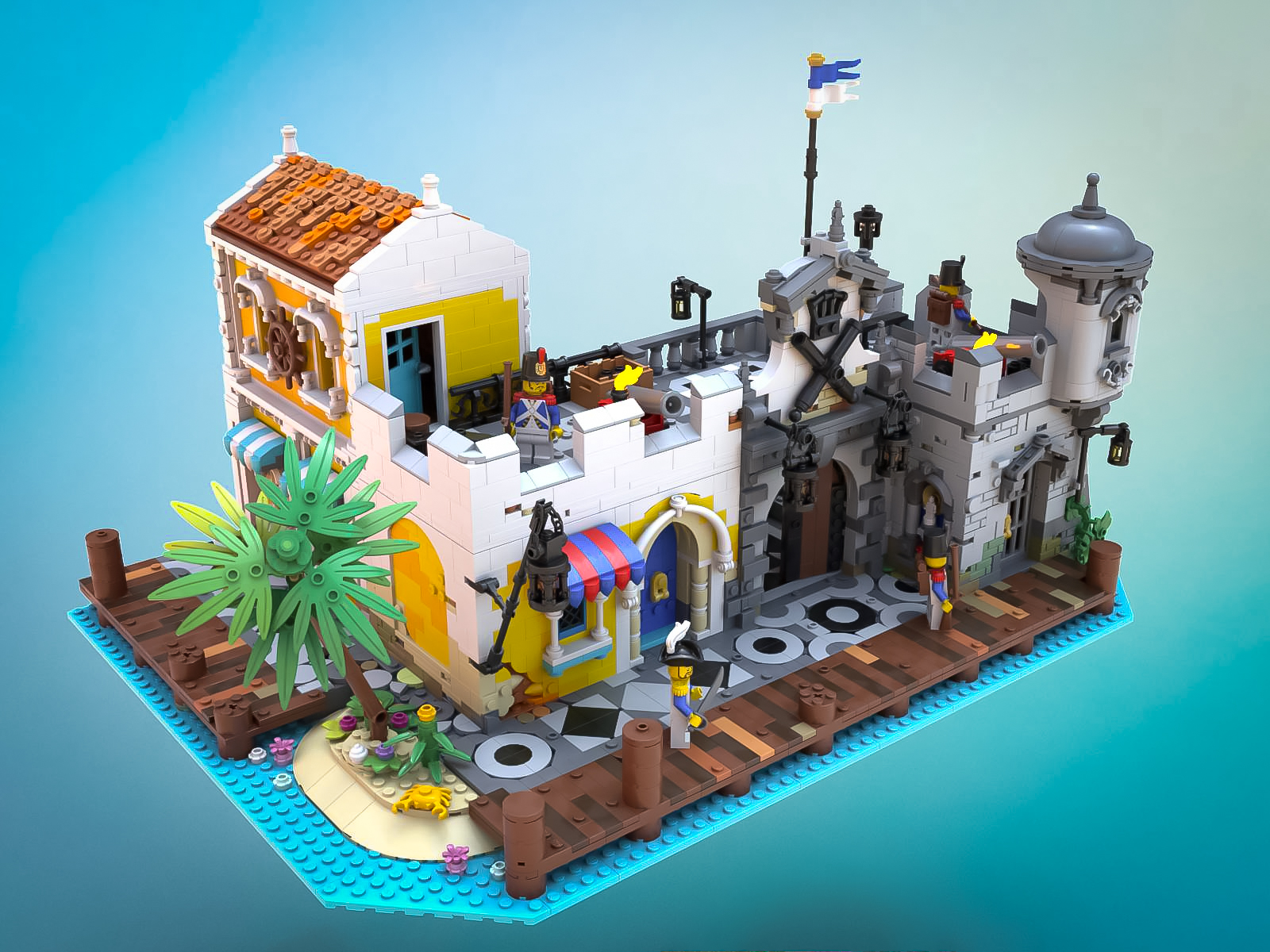The image captures a detailed and well-constructed Lego set featuring a pirate-themed structure that blends elements of a medieval castle with a shop front. The entire scene is set against a light blue to turquoise backdrop, simulating an aquatic environment. The main part of the Lego structure is built on a large, light blue platform that resembles water, while the castle-like building uses mostly white bricks with accents of gray and a roof that is brown and red. 

Dominating the scene is a two-story structure with a circular outpost on the right and a brown walkway that lines both sides of the castle. A characteristic castle door with gating enhances the medieval aesthetic. At the front of the building, a dock extends from the left to the right side, and a man stands on it brandishing a cutlass. The surrounding scene is lively, featuring several Lego figures in what appear to be British naval uniforms standing guard on top of the castle. On the left side of the structure, a palm tree and a tiny yellow crab add to the vibrant details of the set. A patterned sidewalk further completes the realism. At the very top, a flag waves, adding a final touch to this elaborate Lego creation.